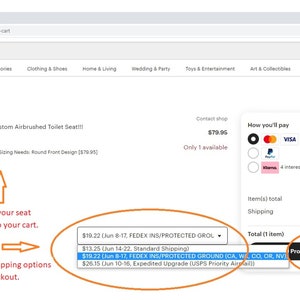**Detailed Caption:**

The image is a screen capture from a website page showing various elements and sections. 

At the top of the image, a continuous gray rectangle spans the entire width of the page. Directly beneath it, there is a lighter gray rectangle, also extending the full width. On the far left side of this rectangle, the word "cart" appears in lowercase black letters. Below this header, there is another light brownish-gray rectangle stretching across the page.

Proceeding downwards, there are several tabs organized horizontally. None of the tabs appear to be selected. The first tab is partially cut off, displaying only the letters "O-R-I-E-S." Moving right, the subsequent tabs are labeled "Clothing and Shoes," "Home and Living," "Wedding and Party," "Toys and Entertainment," and "Art and Collectibles." Beneath these tabs, there is a dividing line followed by a blank white space.

On the left side of the screen, a description reads "T-O-M airbrush toilet seat!!!” Below this, partial text appears, indicating "needs round front design, $79.95." Further down, a half arrow pointing upwards in yellow and the word "Our seat" in red are visible. Following this, "your cart" is displayed, beneath which another yellow arrow points to the right. Below this arrow, the text "P-P-I-N-G options" appears, along with "K-O-U-T."

This right-pointing arrow leads to a circled drop-down box highlighted in a yellow-orange oval. Inside the drop-down, it says "$19.22 (June 8th through 17th, FedEx, INS, protected, G-R-O)." Beneath this, three shipping options are listed: $13.25, $18.22, and $25.15, with the second option highlighted in blue.

On the right side of the page, beginning around the middle section after the blank space under the tabs, an option labeled "Contact Shop" is visible. Below this, the price of $79.96 is indicated, and it states "only one available." To the right of this information, within a outlined rectangular area labeled "How you'll pay," there are three payment options: 

1. The first option shows MasterCard and Visa symbols, next to a black circle with a smaller white circle inside it on the left.
2. The second option to the right features the PayPal logo beside the outline of a white circle.
3. The third option displays a logo in pink with black writing, presumably for Klarna, alongside another white circle outline.

Under all the payment options, the image lists "items total," followed by "shipping," and finally "total one item."

This structured layout captures the intricate details presented on the screen capture of the website page.